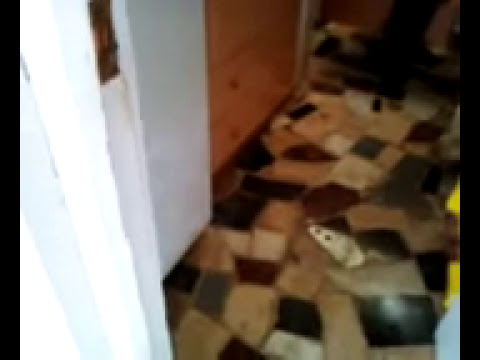This image depicts the interior of a building featuring a distinctive 1960s-style mosaic tile floor. The floor is adorned with an array of tiles in various colors including brown, tan, orange, green, black, beige, and gray. These tiles come in multiple sizes and geometric shapes such as squares, rectangles, triangles, and hexagons, all pieced together in a seemingly uniform yet chaotic pattern. The floor is glossy, though the entire image has a noticeable blur. 

To the left, a wooden wall leads to a white rectangular piece, likely part of a door frame or wall section. Extending from the right side of the image is a small, sideways, yellow triangle. The mosaic floor appears to angle downward at approximately 45 degrees. In the background, there is a hint of what looks like a wooden chest or cabinet amidst some potential clutter, adding complexity to the scene. The room has white walls, contributing to a somewhat muddled yet intriguing visual composition due to the overall blur of the photograph.